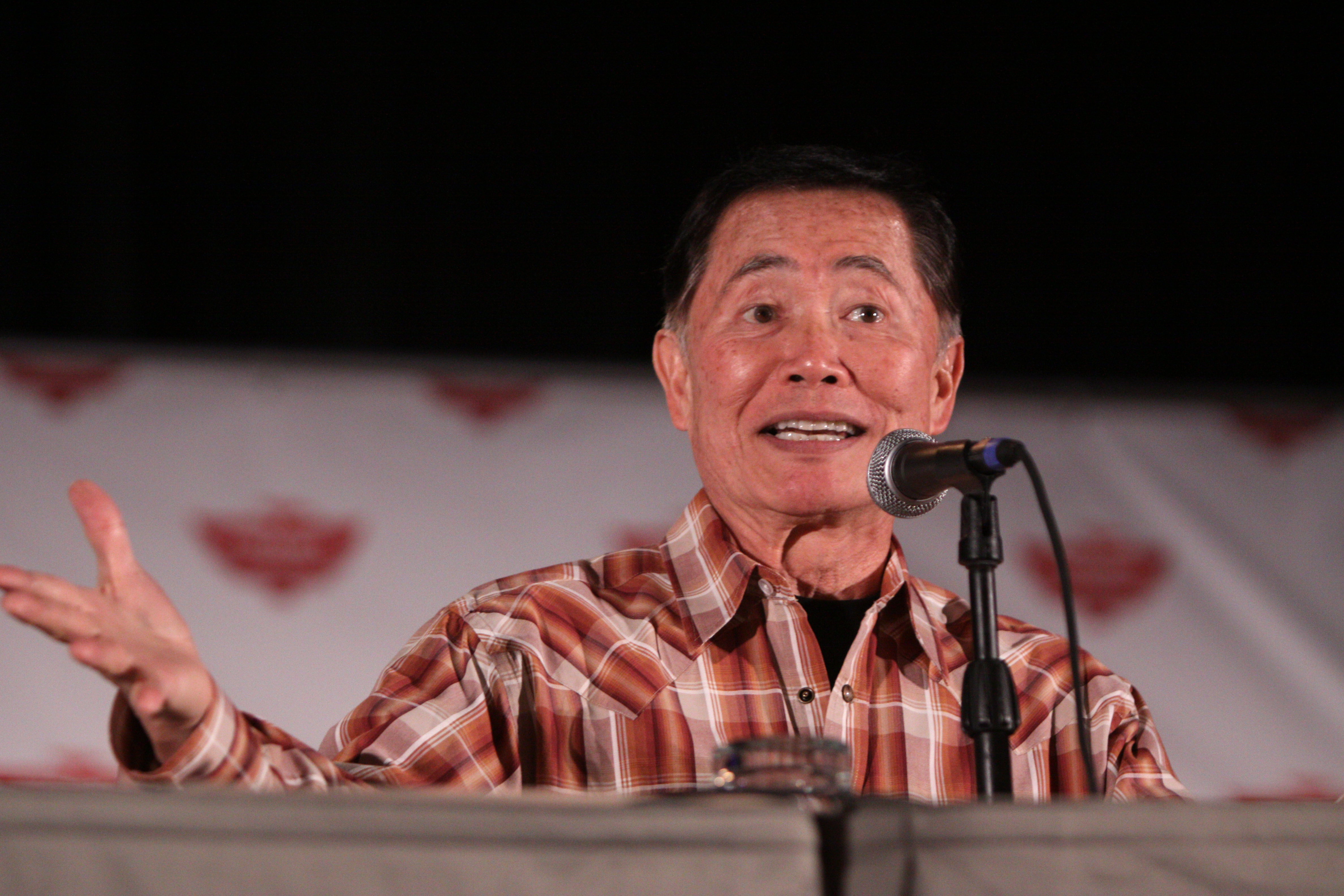This detailed image captures an elderly Asian man seated at a table or podium, speaking into a microphone. The microphone features a black stand with a silver ball at the front, and has a small piece of blue on it. The backdrop behind him is predominantly black on the upper half, with a white section displaying red logos that could be heart, bird, or butterfly-shaped.

The man has distinctive features, including age spots, black hair with gray sideburns, shiny skin, big ears, and a wide mouth. He is dressed in a shirt with an undershirt visible beneath it. His right arm is extended outward with his hand open in a gesturing manner, as his mouth is open mid-speech. In front of him sits a glass of water on a dark slate gray table.

The scene appears color-coordinated with shades of black, burnt orange, cream, white, brown, and dark slate gray. His demeanor and the micro-movement captured suggest he may be addressing an audience, although his eyes look slightly to the right of the camera. It's unclear whether this image was taken indoors or outdoors, or during the day or night, adding a layer of mystery to the moment captured.